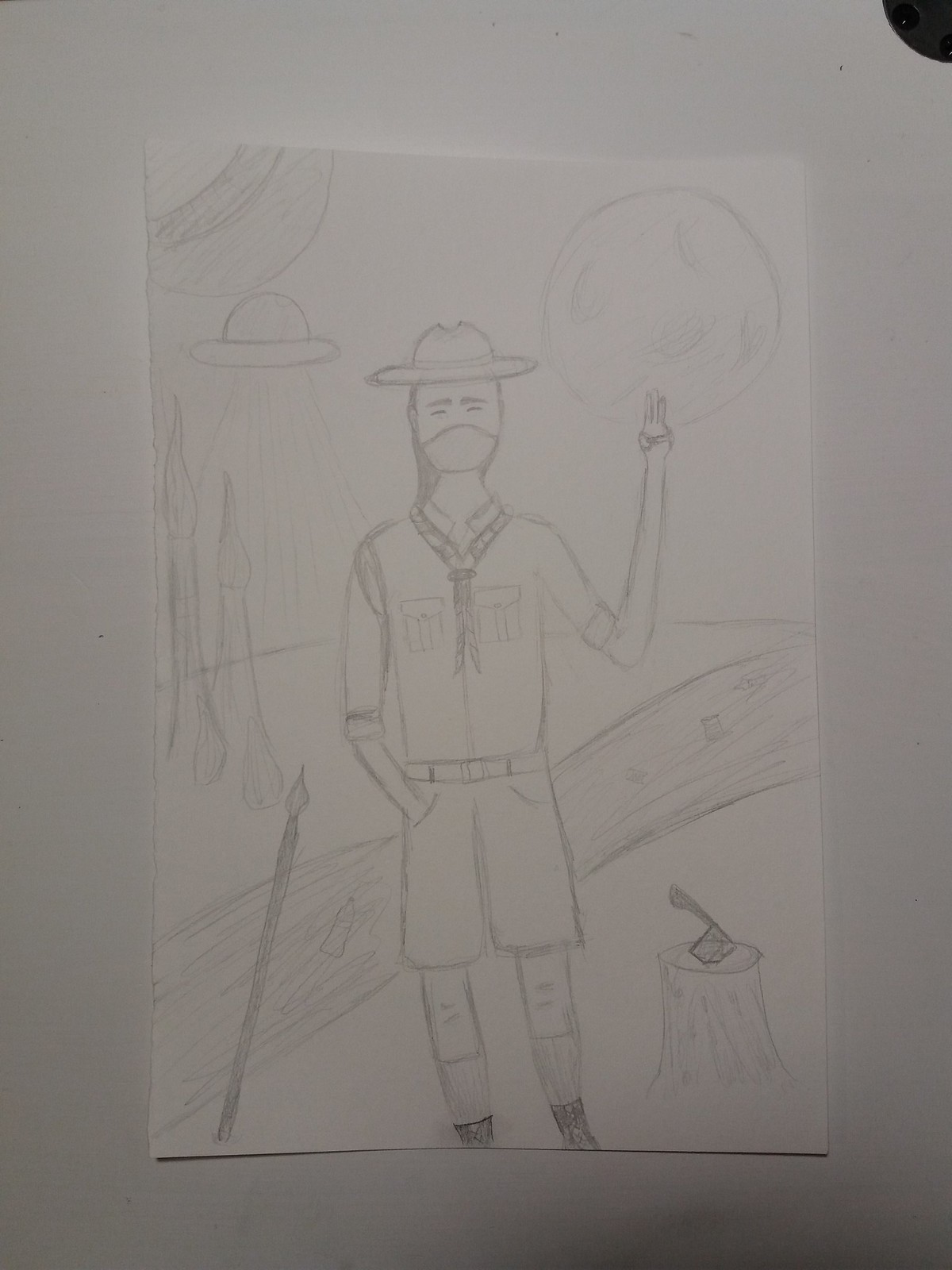A detailed pencil drawing on a white sheet of paper is prominently displayed at the center of this photograph, which rests on a white surface. In the upper right corner of the image, a section of a black circle is visible, mostly cropped out, showing just a small triangular portion against the stark white background.

The drawing appears to be done by an amateur artist, possibly a teenager, and depicts a scene featuring a man in a Boy Scout uniform complete with a hat, scarf, and classic attire. The man is positioned slightly to the left on the paper, raising his left arm towards the moon, his hand forming a Scout salute with three fingers extended. In the night sky behind him, a UFO adds an element of mysterious intrigue.

On the ground behind the man, there is a felled log and a tree stump, from which an axe protrudes, suggesting a recent wood-chopping activity. The attention to detail, despite the artist's apparent lack of professional training, captures a unique narrative blending elements of scouting, wilderness, and extraterrestrial wonders.